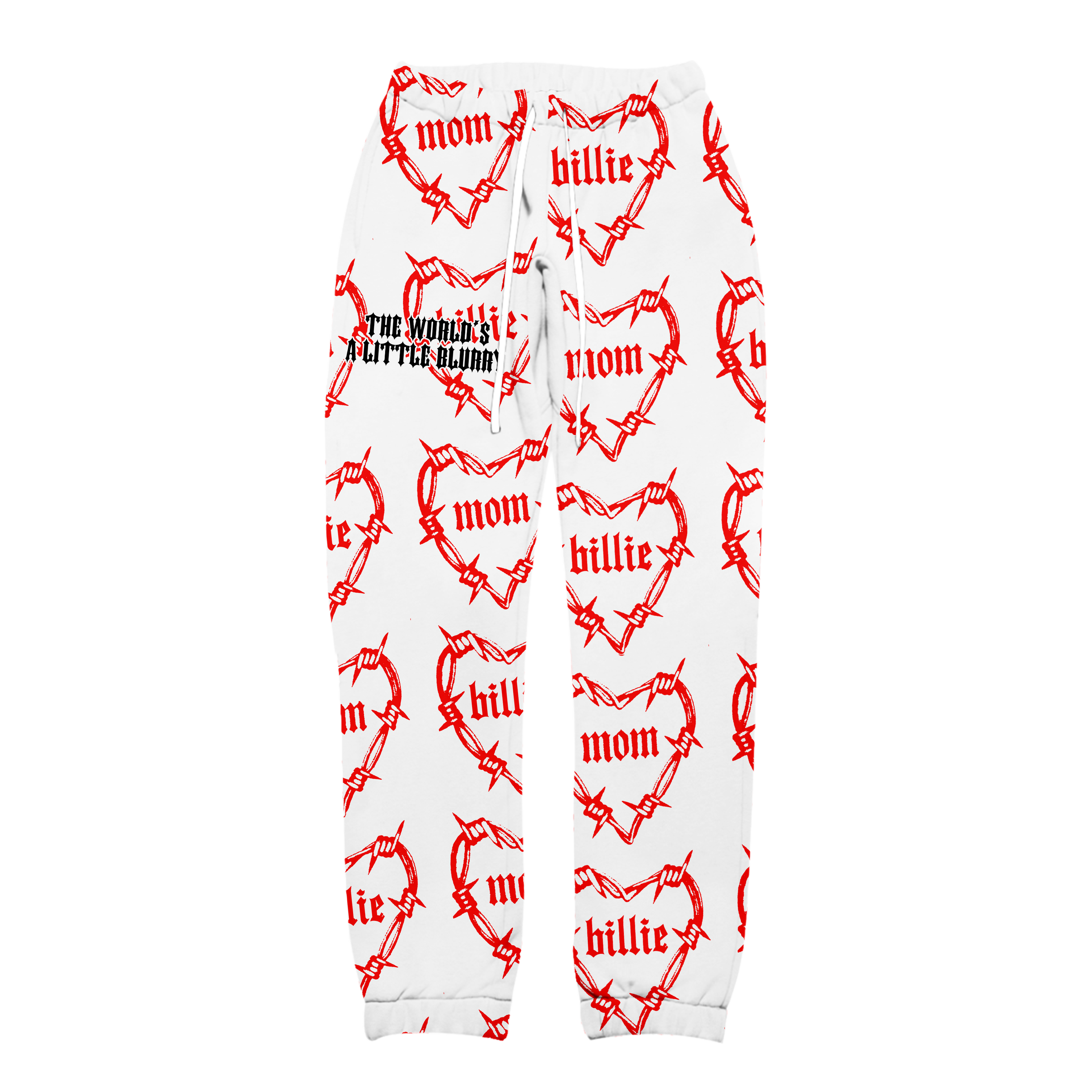This image is a close-up shot of a pair of white sweatpants, likely concert merchandise, featuring a seamless pattern of red hearts designed to look like barbed wire. Some of the hearts contain the words "Mom" and "Billie" in gothic font. The sweatpants have black text on the upper left thigh that reads, "the world's a little blurry." The pants are jogger-style with an elastic waistband, complete with two white drawstrings, and elastic cuffs at the ankles. The photograph has a transparent background, possibly suggesting it's intended for a catalog or website display.